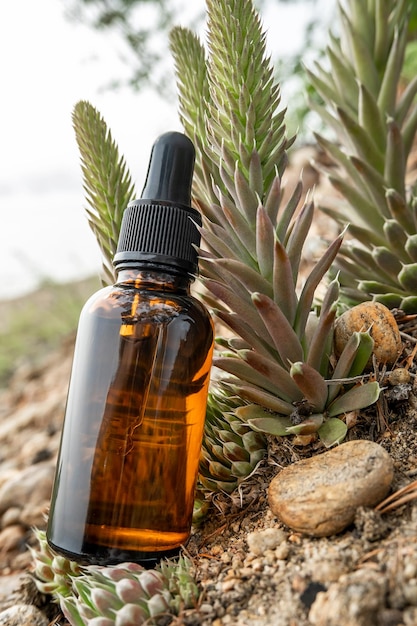This image showcases a close-up of a small, dark brown glass bottle with a black plastic screw-on squeezer bulb attachment, commonly referred to as a dropper bottle. The dropper tube is visible inside the bottle, which appears to contain a clear liquid. The bottle is centrally positioned, sitting atop a mixture of gravel and rocks. Surrounding the bottle are various succulent plants, including a tall, colorful green cactus with prickly tips, and a smaller cactus positioned just beneath the bottle. The backdrop reveals a cloudy sky, more greenery, and a flat terrain of dirt, contributing to the natural outdoor setting. The composition suggests the bottle might contain an extract from one of the plants, potentially for medicinal or cosmetic use.